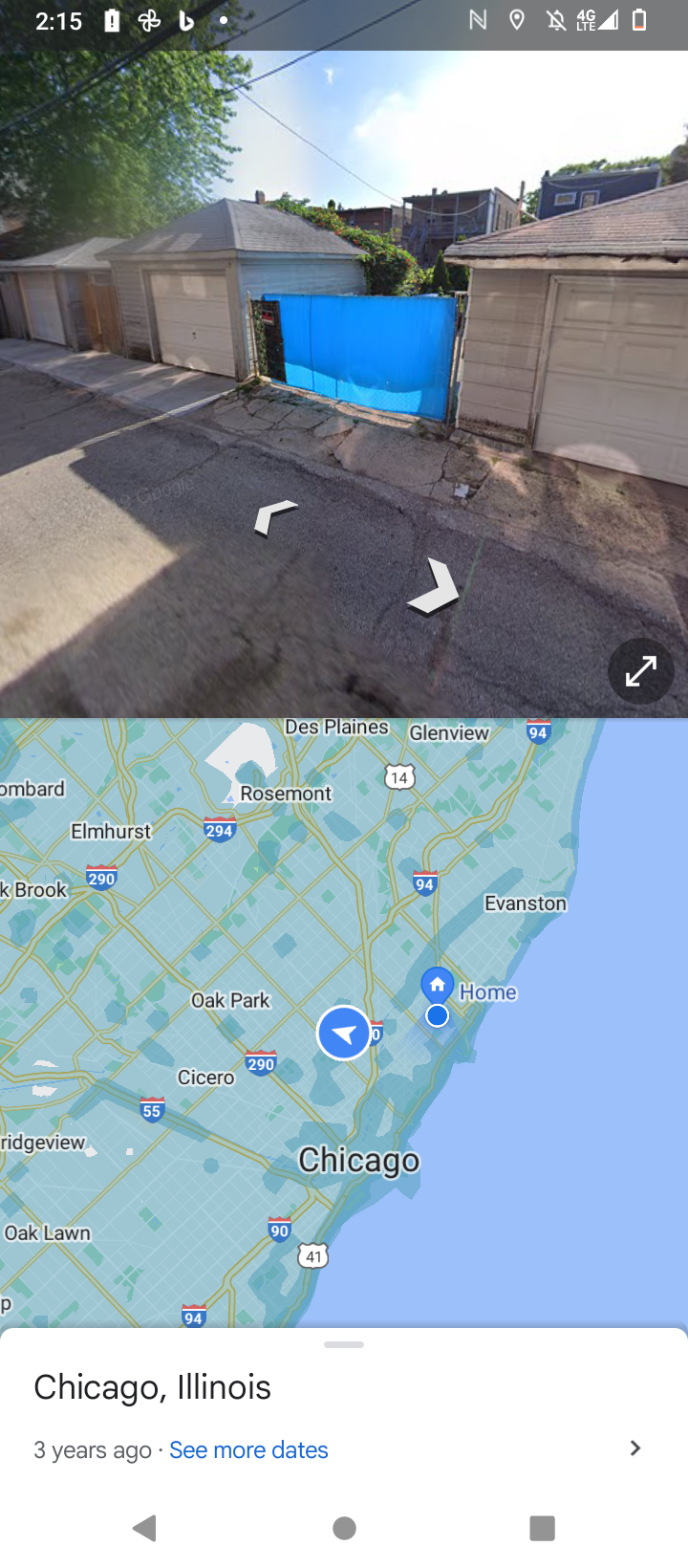This image appears to be a screenshot from a smartphone displaying two distinct sections. The upper part shows a sequence of standalone garages which appear to be positioned along a gray asphalt driveway or road. Notably, there is a gray garage with a white door on the left, followed by a conspicuous blue tarp in the center, and then additional garages. The blue tarp is particularly prominent, situated right in the middle of the image. In the upper left corner of the image, the number "215" is displayed in white font. Adjacent to this, there are several status icons: a battery indicator, a signal icon, a lowercase "b," a dot, and other typical smartphone status symbols—including what seems to be a map marker, an icon with a line through it, a sideways triangle perhaps representing cell service, and a battery indicator. Additionally, two white arrows at the bottom of this section suggest the presence of more images that can be viewed by clicking through.

The lower part of the screenshot displays a map focusing on the Chicago, Illinois area. This map clearly outlines several highways and includes multiple city labels. Beneath the word "Chicago," it indicates "three years ago," suggesting a historical view. In blue text below this, the phrase "See more dates" offers the option to explore additional time frames. This bottom section appears to be a time-stamped map view, likely presented within a mapping or street view application, allowing users to select specific locations and dates for contextual road views.